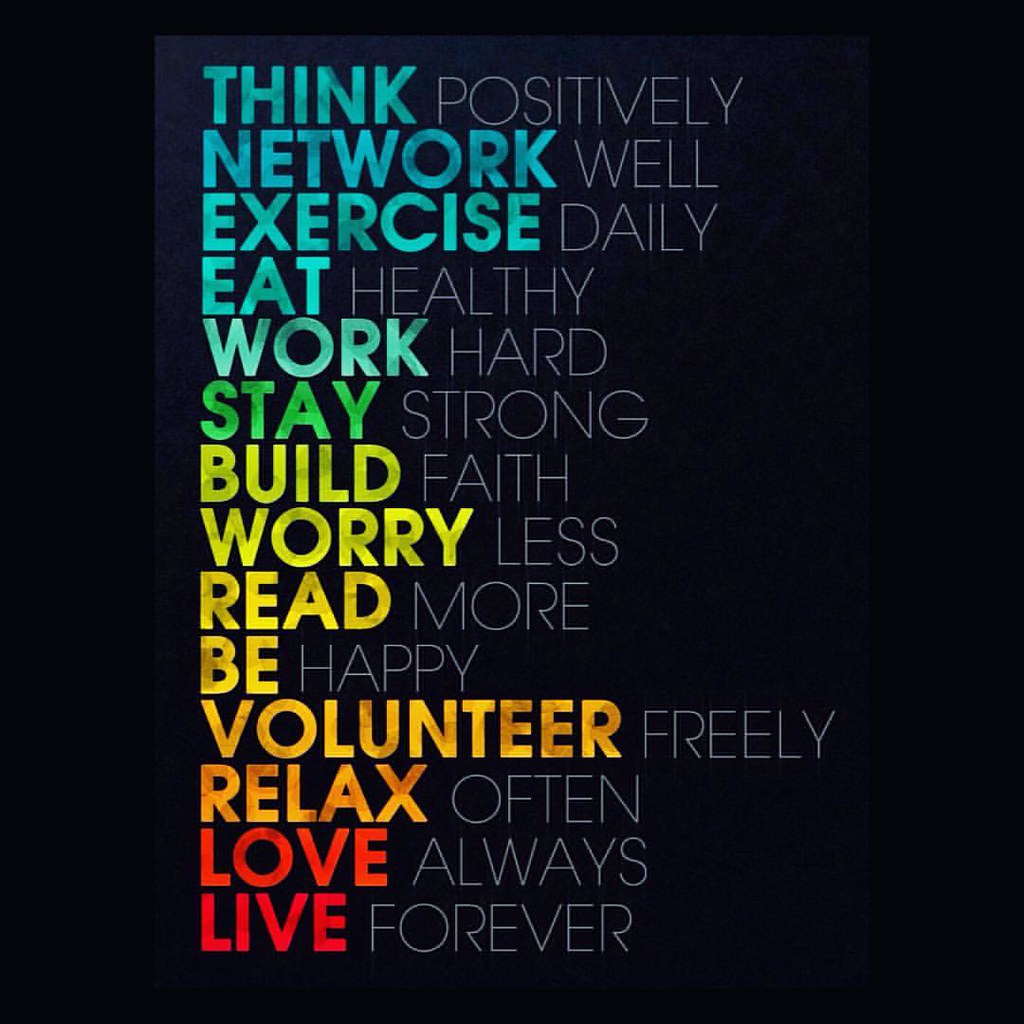The image is a motivational poster featuring text centered on a dark navy blue gradient background that subtly transitions from darker at the bottom to lighter at the top. The poster displays an array of motivational phrases, each comprising two words with the first word in bold, colored capital letters and the second in thinner, white capital letters. The words "think," "network," "exercise," "eat," and "work" are in various shades of blue, "stay" in green, "build," "worry," "read," "be," and "volunteer" in yellow, "relax" in orange, and "love" and "live" in red. The complete text reads: "THINK POSITIVELY, NETWORK WELL, EXERCISE DAILY, EAT HEALTHY, WORK HARD, STAY STRONG, BUILD FAITH, WORRY LESS, READ MORE, BE HAPPY, VOLUNTEER FREELY, RELAX OFTEN, LOVE ALWAYS, LIVE FOREVER." The words are consistently structured with the first word in bold color and the following word in thin white, all capitalized, creating a stark, inspiring display against the dark background.